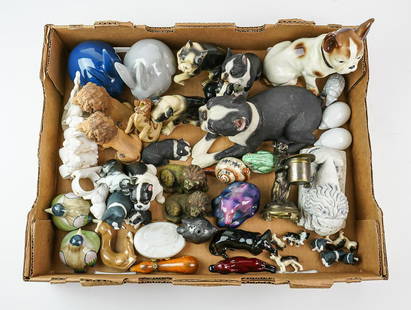The image depicts a shallow cardboard box, set against a gray background, brimming with an assortment of small, intricately crafted figurines, likely made of porcelain or sculpted clay. Dominating the ensemble are various animal figures, including at least twelve small dog statues resembling Boston Terriers, some of which are black and white, with one notably larger brown and white figure situated in the upper right corner. Additionally, the collection features two meticulously painted and glazed bunny rabbits, two small lion carvings, and several types of birds such as geese or ducks. There is also a unique snail figurine and potentially some sea creature representations among the assortment. The array of detailed trinkets scattered within the box suggests they were created in a craft environment, highlighting the delicate artistry involved in their painting and glazing.